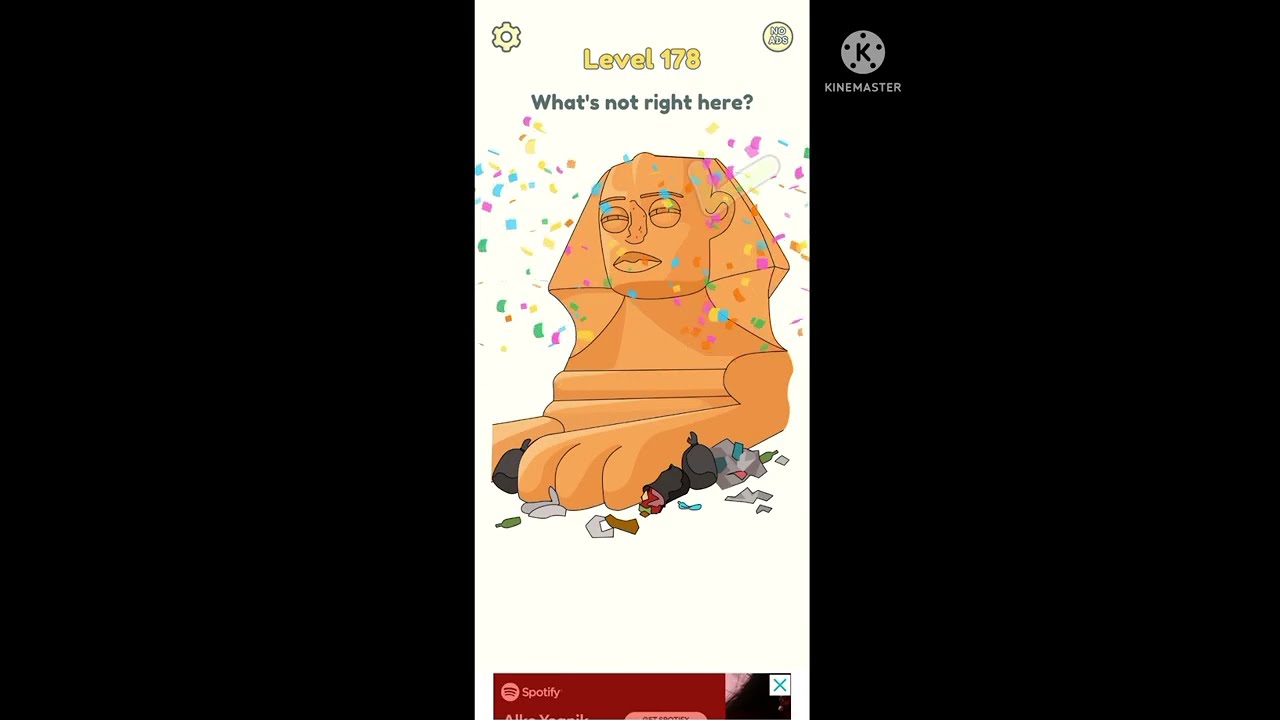In the center of a horizontally rectangular image with solid black borders on both sides, there is a vertically oriented, stylized drawing resembling a cartoonish sphinx. This central figure depicts a humanoid face with slightly open eyes and eyebrows, seemingly wearing a hood-like garment draped over its head. The color of the character is predominantly brown, interspersed with floating specks of blue, purple, and yellow, mimicking confetti. Extending from the shoulders and chest are disproportionately large hands that reach out towards the viewer, while the base of the figure features lion-like paws and is surrounded by some apparent garbage. At the very top of the white background, "level 178" is written in yellow letters. Directly below this, in blue letters, is the question, "what's not right here?" with a question mark. Additionally, a small part of another screen with a red background bearing the word "Spotify" is visible at the bottom of the central image.